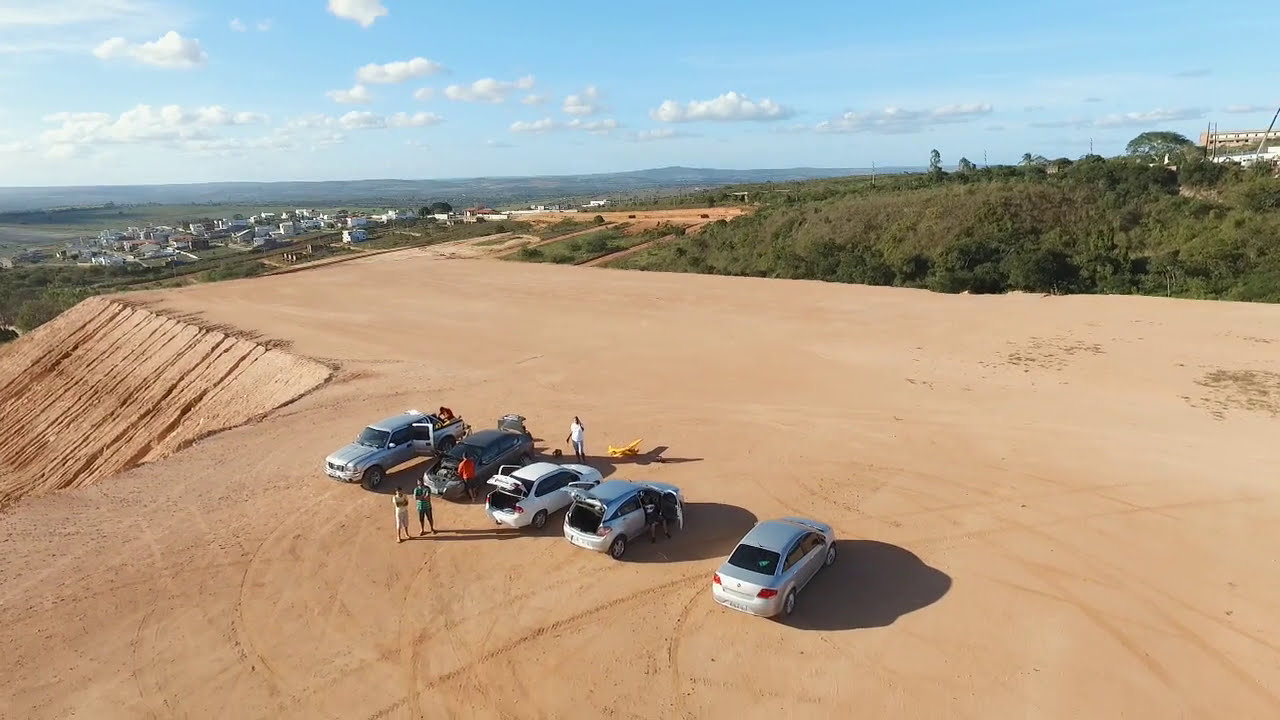This aerial photograph, likely taken from a drone or a high vantage point, captures a flat, reddish, crushed brick-like sandy plateau. On this plateau, five cars are prominently lined up diagonally from right to left. The first car on the right is a silver sedan, followed by a silver hatchback with its trunk and door open. Next is a white hatchback with its trunk open, then a dark-colored car with its trunk open, and finally, on the leftmost side, a silver truck with its doors open. Approximately five or six people are milling around these vehicles, which also share the ground with what seems to be a toy airplane. To the left, the terrain drops off at a roughly 45-degree slope. On the right side of the image, a thicket of trees and greenery is visible. In the far distance on the left, a cluster of buildings—possibly a town or small city—can be faintly seen under the partly cloudy, light-blue sky, which occupies the upper fifth of the photograph. Additionally, even further on the horizon, one can make out a somewhat hilly or mountainous area, adding depth to the scene.